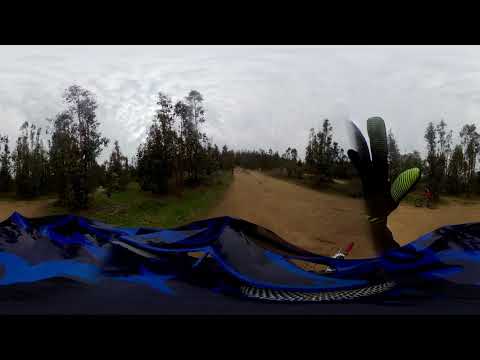In this panoramic, 360-degree image taken outdoors during an overcast daytime, a person rides down a large dirt path amidst a forested area. The rider, visible from a helmet-mounted camera, is likely on a motorcycle or dirt bike, given the gear they are wearing, including a distinctive blue and black helmet and black gloves with yellow fingers. As the rider navigates the path, their right hand is clearly seen gripping the handlebars. The surrounding environment features a dense array of trees, including pine trees, shrubs, and grassy patches, contributing to the lush scenery. Additional pathways can be spotted in the distance, suggesting a network of trails within the area. The image exhibits noticeable distortion typical of a 360-degree capture, creating a slightly warped effect throughout. This effect is most prominent in the middle of the frame, where the dirt path and natural elements appear broken up and exaggerated. The bottom of the image shows some patches of blue, possibly a body of water, though this is unclear due to the distortion and hilly background. Black framing in thick rectangular shapes extends across the top and bottom edges of the photo, adding a dramatic element to the scene.